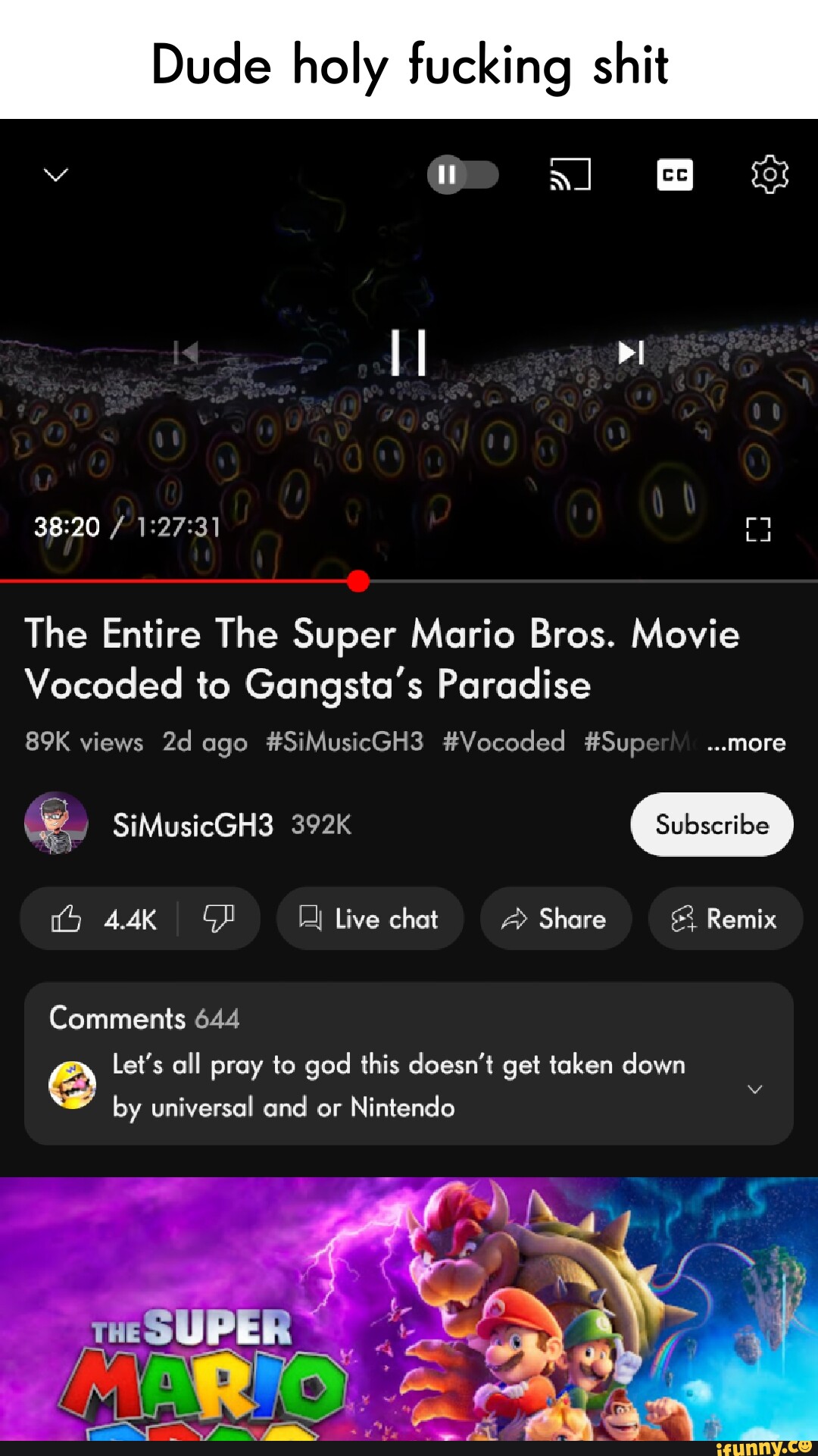**Detailed Description:**

This is a screenshot of a paused YouTube video titled "The entire The Super Mario Bros. movie vocoded to Gangsta's Paradise," which has garnered 89,000 views in just 2 days. The video is currently paused at the 38-minute and 20-second mark out of a total runtime of 1 hour, 27 minutes, and 31 seconds. The paused frame features numerous glowing, smiley faces in a crowd, creating a surreal visual effect. At the top of the screenshot, a comment reads, "Dude, holy fucking shit." Below the video title, there's a plea for the content to remain online, saying, "Let's all pray to God this doesn't get taken down by Universal and/or Nintendo." Additionally, an image of the movie poster for "The Super Mario Bros. movie" is displayed, featuring the cartoon characters Mario, Luigi, Donkey Kong, Princess Peach, and Bowser.